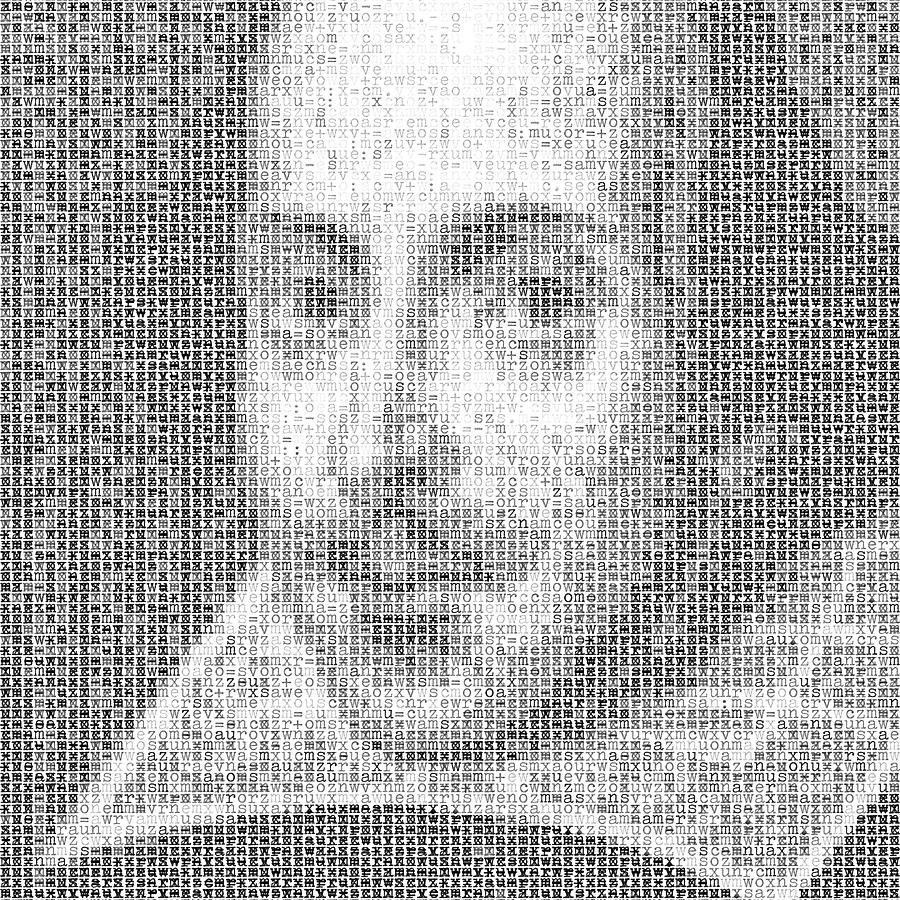In this detailed black and white typewriter art piece, William Shakespeare is depicted in an abstract yet recognizable manner. The image ingeniously utilizes varying shades of text, from light to dark, created by overlapping different letters and special characters from old-style type fonts. The shading technique conveys depth, with denser clusters of text representing darker areas such as his pupils, eyebrows, and hair, while sparser text forms lighter areas like his face. Shakespeare's characteristic features are evident: a thin mustache, dark eyebrows, and dark eyes looking to the right. He is adorned in a dark shirt featuring a prominent white square collar, reminiscent of his iconic attire. The text forming this intricate image ranges from regular letters like W, C, A, X, and Y to more abstract, emoji-like glyphs, creating a mosaic effect. This sophisticated composition not only captures the essence of the renowned historical writer but also showcases the creativity and precision of typewriter art.